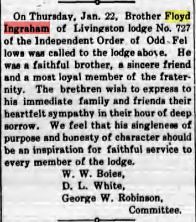The image depicts a small newspaper clipping with a white background and black text, featuring a highlighted word, "Ingram," in red. The text reads: "On Thursday, January 22nd, Brother Floyd Ingram of Livingston Lodge No. 727 of the Independent Order of Odd Fellows was called to the lodge above. He was a faithful brother, a sincere friend, and a most loyal member of the fraternity. The brethren wish to express to his immediate family and friends their heartfelt sympathy in their hour of deep sorrow. We feel that his singleness of purpose and honesty of character should be an inspiration for faithful service to every member of the lodge." The notice is signed by W. W. Bowles, D. L. White, and George W. Robinson Committee.